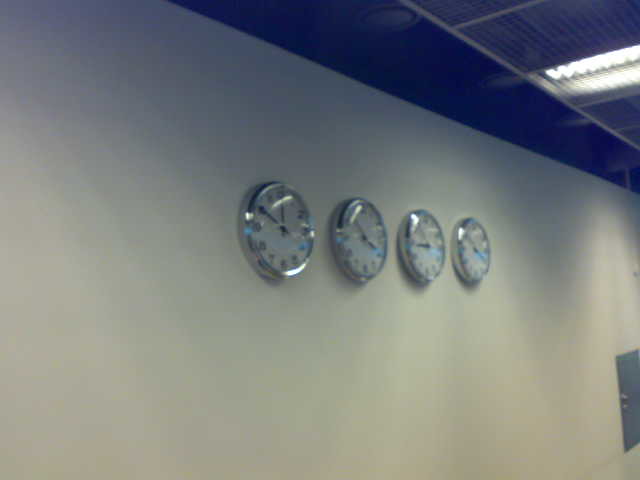This photograph captures a slightly grainy scene featuring four silver-bodied clocks mounted in a row on a pristine white wall. Each clock showcases a white face with dark-colored hands and black numerals, and the glass coverings on the clocks reflect light subtly. A hint of ceiling is visible above, exhibiting a metallic look that adds a modern touch to the setting. On one side of the frame, a small, silver door is discernible on the white wall, giving a hint of functionality. The sunlight streams in through the ceiling, playing with shadows against the wall and lending a murky, atmospheric effect to the overall composition.